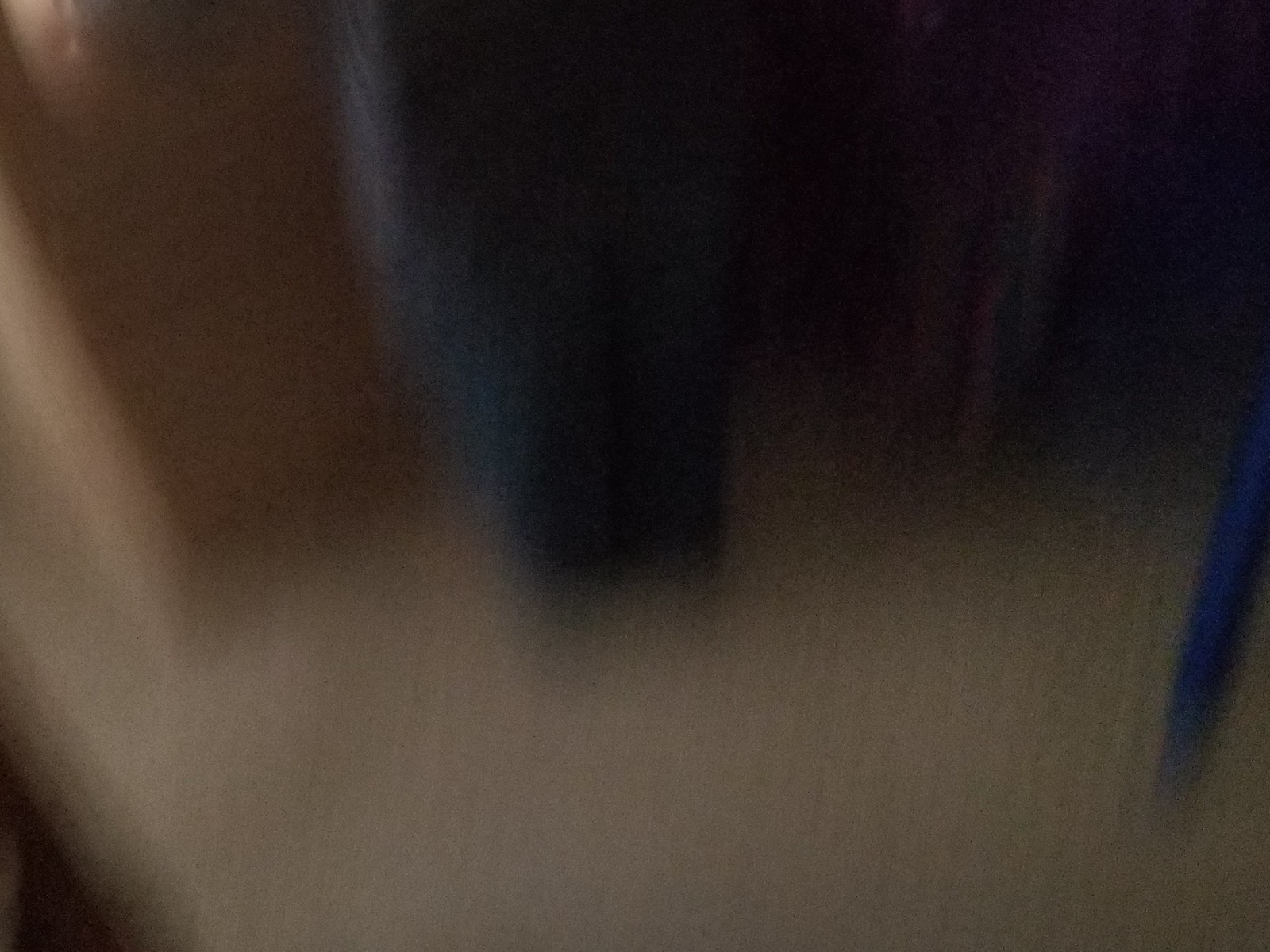A highly out-of-focus image is presented, rendering the scene nearly indistinguishable. In the center, there is a blurry blue blob, while to its right appears a similarly obscured purple area. On the far right, a streak of blue, possibly the slender leg of a chair or table, is somewhat discernible. The bottom portion, likely the floor, is entirely white. From the upper left corner extending to the middle left side, a faint brown rectangular shape can be vaguely identified, though details remain elusive due to the blurred quality of the photograph.